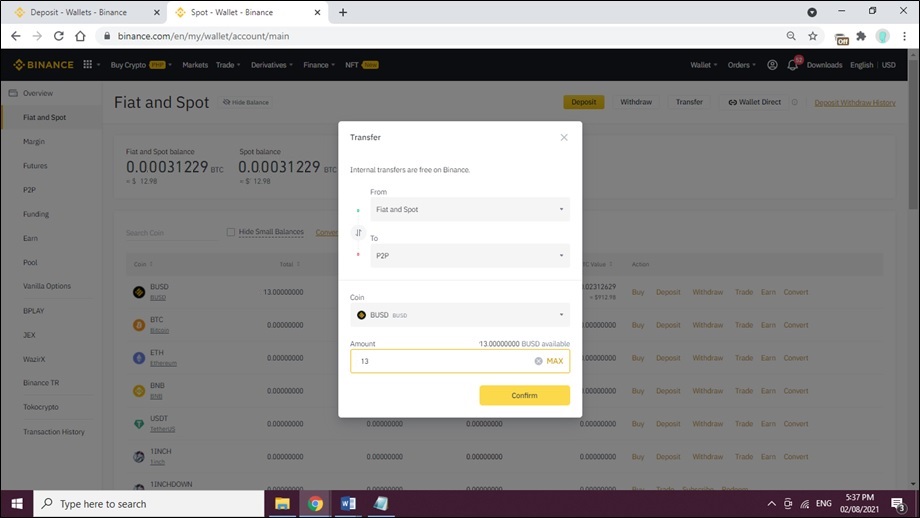This image showcases the Binance website open in a desktop browser with two tabs visible at the top left corner. The active tab displays "Spot, Wallet, Binance," while the other tab reads "Deposit, Wallet, Binance." 

At the top of the webpage, a black banner displays the Binance logo on the left, followed by navigation options labeled "Buy Crypto," "Markets," "Trade," "Derivatives," "Finance," and "NFT." On the right side of the banner are links to "Wishlist" and "Orders," alongside an account icon, an alert icon with a red notification dot, download options, language selection set to English, and currency set to USD.

The main body of the page, set against a white background, features an overview index on the left with vertically-arranged categories. Dominating the top of the page is the heading in bold black letters, "Fiat and Spot." A central pop-up titled "Transfer" commands attention, with a bright yellow "Confirm" button at the bottom of the pop-up box. This detailed visual provides a comprehensive look at the user's interaction with the Binance platform.